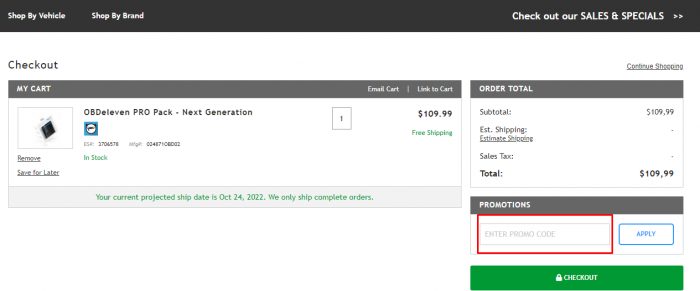This screenshot captures a checkout page of a website featuring a sleek and user-friendly design. At the top of the page, there is a prominent black banner with navigational options. On the left side of the banner, in small white letters, it says "Shop by Vehicle." Right next to it, the text "Shop by Brand" is also displayed in small white letters. On the far right, the banner features "Sales and Specials" in slightly larger white letters with two white dots immediately to the right.

The page's body has a clean white background. On the far left side, the word "Checkout" appears in gray letters, indicating the current page. Below this, there is a box with a gray banner at its top. On the left side of this gray banner, the words "My Cart" are prominently displayed. Towards the right side of the banner, there are options for "Email" and "Link to Cart."

The main section of the cart box shows an item that has been added. The thumbnail image of the item appears on the left side, with the name and description of the item to its right. Just beside this description, a small gray box indicates the item quantity, currently set to one. On the far right of this section, the item's price is displayed, and directly below it, "Free Shipping" is highlighted in blue text. Beneath the thumbnail image of the item, there are two clickable options: "Remove" and "Save for later."

To the right of this cart section, there is a smaller box summarizing the order totals. Inside, it lists the subtotal, shipping, sales tax, and a bold "Total" amount. Underneath this box, there is a smaller section labeled "Promotions." Within this section is a box to enter a promotional code, which has been edited with a red triangle overlay concealing the code input area.